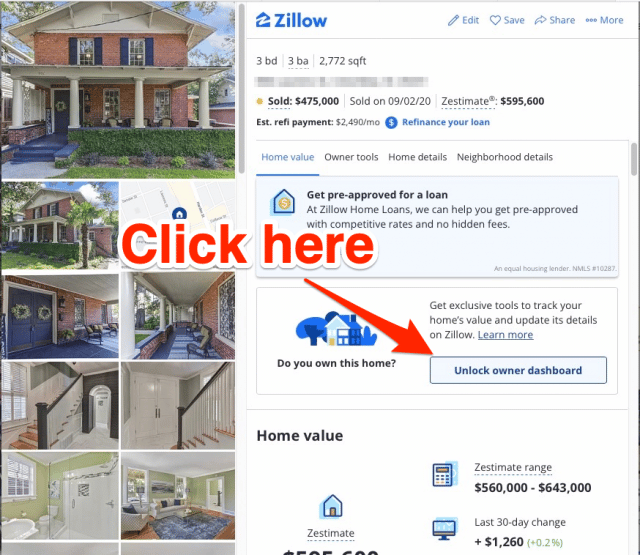Title: Detailed Zillow Property Listing Overview

Caption: 

This detailed webpage from Zillow displays property listings with various interactive features. On the left side of the page, a prominent red-brick building with white signage and roofs is visible. To the right, the iconic Zillow logo, depicted in either green or blue, is showcased with the text "Z-I-L-L-O." Below the logo, a white rectangle provides critical property details: "3BD" (3 Bedrooms), "3BA" (3 Bathrooms), and a total area of 2,772 square feet. Both the bedroom and bathroom indicators are underlined, suggesting that these elements are clickable and likely lead to additional images or information.

Adjacent to the logo, the top right corner features several functional icons: a pencil labeled "edit," a heart marked "save," an arrow for "share," and a set of three ellipses indicating more options. An orange circle, also underlined and clickable, indicates the property's sold status with the caption "Sold $475,000" and the sale date "09-02-20" (September 2nd, 2020). Notably, the current estimate is boldly displayed as "$595,600."

Below the main information, additional images of the property are laid out, including a side view and a front view of the house, which boasts striking big blue doors and a white banister. Further, interior shots reveal a bathroom designed with white and steel green tones. A red arrow marked "click here" directs users to unlock the owner dashboard, enhancing the interactive experience.